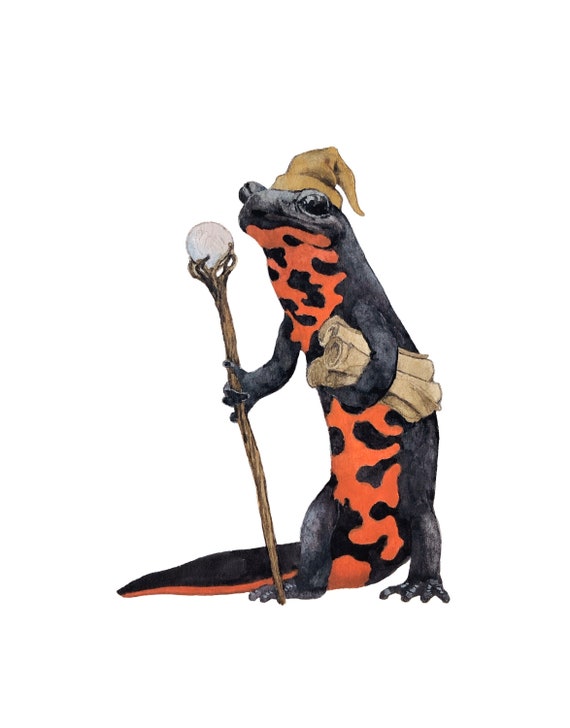The image depicts a detailed drawing or statue of a salamander, standing upright on its hind legs. This magical creature is dressed like a wizard, evoking imagery akin to Gandalf from Lord of the Rings. The salamander's skin is primarily dark gray to black, with an underbelly adorned with irregular orange and red splotches that extend to the underside of its tail. It holds a wooden staff in its right hand, topped with a white orb that reaches almost to the creature's face. In its left arm, it carries three or four off-white scrolls. Adding to its wizardly appearance, it wears a pointed gray hat that hangs down in the back. The salamander's calm, neutral eyes gaze slightly off to the side, reinforcing its thoughtful and mystical demeanor.